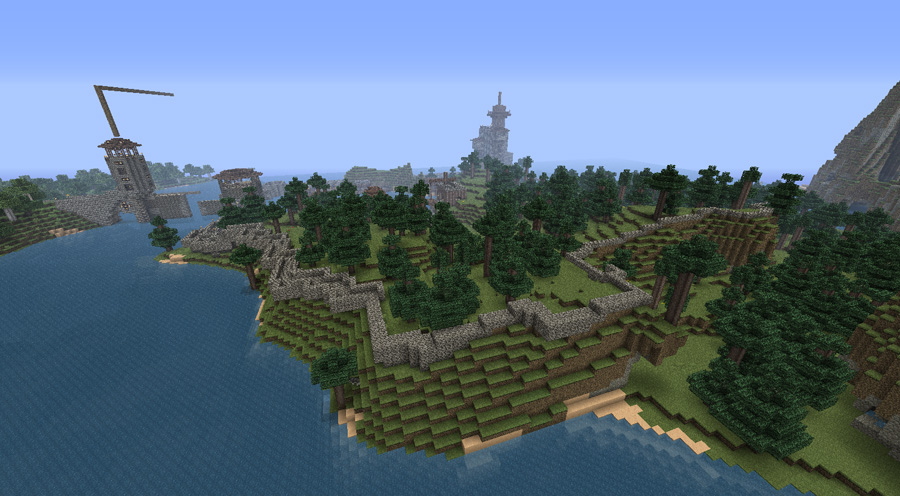The image depicts a highly detailed, artificial landscape that appears to be constructed from Lego-like or pixelated blocks, reminiscent of a Minecraft scene. Dominating the scenery are lush green areas populated with numerous dark green, pine-like trees. A significant body of blue water occupies the left portion of the image, contrasting with the staggered, terraced grassy sections that look like steps made from blocks. In the background, there are intricately detailed stone buildings and structures, including a small tower with an antenna-like pole poking into the sky and a zigzagging gray wall resembling an old fort. On the far right, a gray mountain extends high above the landscape. The entire scene exudes a detailed, blocky aesthetic, creating an impression of a virtual seaside village.